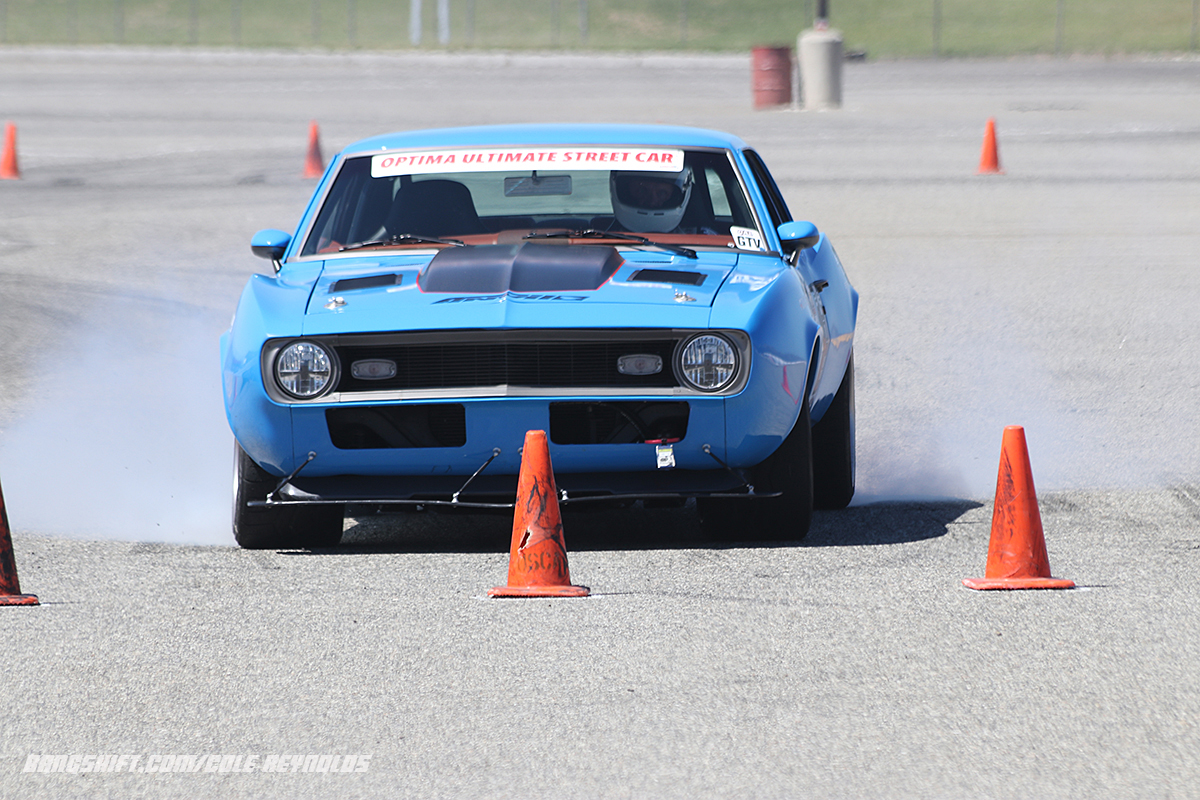The image captures a dynamic scene of a light blue 1968 Chevrolet Camaro navigating through an obstacle course on a gray pavement surrounded by green grass. The photo, taken from a slightly elevated vantage point without showing the sky, features the car prominently in the center, facing towards the viewer. The Camaro has a distinctive black middle scoop on its hood and a white banner across the top of the windshield that reads "Optima Ultimate Street Car" in red letters. The driver, wearing a white helmet, appears focused as white smoke billows from the tires, indicating a sharp maneuver. Scattered around the car are several orange plastic cones, some with visible dark markings and scratches, suggesting frequent impacts. The cones are arranged in a spaced-out pattern that forms a challenging route for the vehicle. The bottom left corner of the image bears the text "bangshift.com / Cole Reynolds."